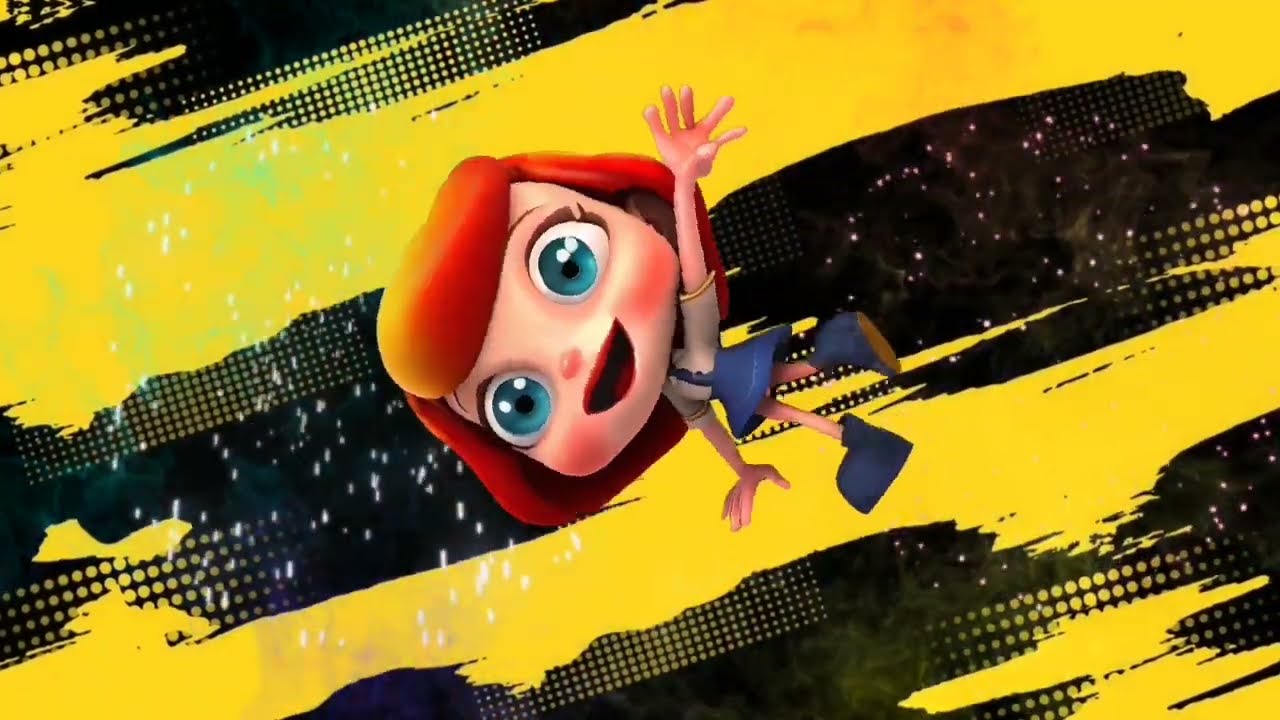The image depicts an animated cartoon girl with an oversized square head, medium-length red hair, and large bluish-green eyes. She has pale skin, rosy cheeks, and an open mouth displaying her gums in a cheerful smile. The girl, dressed in a white top and blue skirt, with large blue shoes, stands slightly turned to the left, with her head facing the left and her feet to the right. She has one arm extended outward as if waving, while the other rests by her side. The background is a mix of varying shades of yellow and black with smoky green or purplish streaks, giving an impression of seeing through outer space or the Milky Way. This setting is adorned with scattered white dots, enhancing the floating, dreamy essence of the scene, and the entire artwork appears to be a digital piece, possibly from a game.